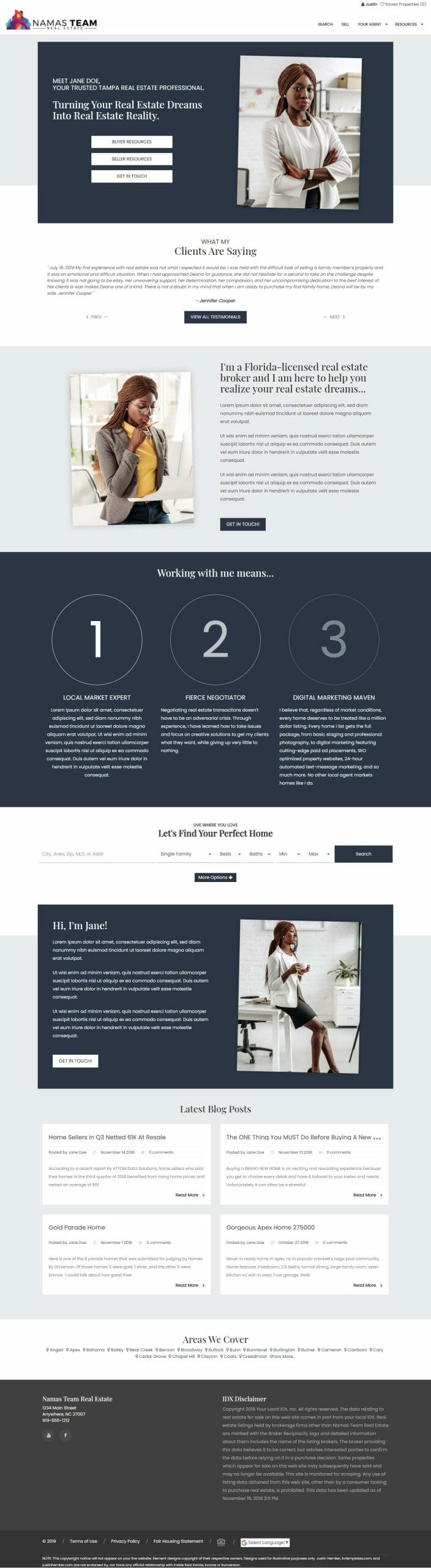This screenshot showcases a detailed section of the NAMAS Team Real Estate website, prominently featuring the professional profile of Jane Doe, a dedicated real estate broker based in Tampa, Florida. 

In the upper left-hand corner of the page, the website's title "NAMAS Team Real Estate" is clearly displayed next to a vibrant logo depicting an architecturally stylized home, rendered in a watercolor palette. 

The first banner on the page introduces Jane Doe as "your trusted Tampa real estate professional," featuring a mission statement to turn clients' real estate dreams into reality. Below this heading are three action buttons labeled “Buyer Resources,” “Seller Resources,” and “Get In Touch.” To the right of these buttons, a professional photograph of Jane Doe shows her standing confidently with her arms crossed, dressed in a white suit and shirt.

Further down the page, a section titled "What my clients are saying" presumably contains client testimonials, though the small text was difficult to read in this screenshot. A prominent blue button labeled “View All Testimonials” encourages visitors to explore more feedback from Jane's clients.

Another banner highlights Jane's credentials with the statement, "I'm a Florida licensed real estate broker, and I'm here to help you realize your real estate dreams," paired with another thoughtful image of Jane in a contemplative pose.

The page continues with extensive information about Jane, including a personalized greeting, "Hi, my name is Jane," and additional images of her. It also features links to her blog posts, details on the areas she covers, and other relevant real estate resources, making it a comprehensive and informative web page dedicated to her professional services in real estate.